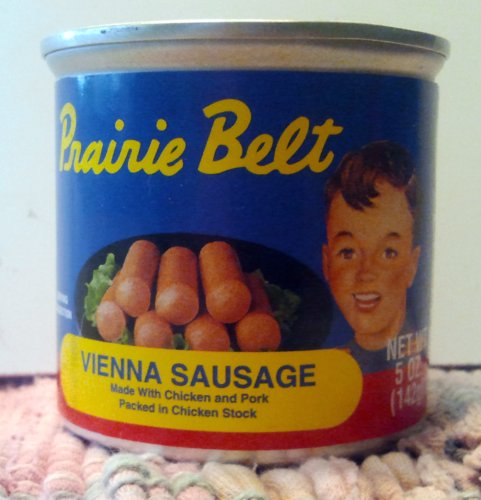This image is a close-up photograph of a small, round silver can of Vienna sausages against an off-white background. The product, Prairie Belt Vienna Sausage, is prominently displayed with a detailed label. The label features a blue background with "Prairie Belt" written at the top in yellow cursive letters. Below this, there is an illustration of a 1950s-style boy with freckles and a partial smile looking towards a black, round plate in the center of the label. On the plate, there are two rows of Vienna sausages, stacked one over the other. A yellow horizontal banner beneath the plate has red lettering that reads, "Vienna sausage made with chicken and pork, packed in chicken stock." The overall color scheme of the label includes blue, yellow, and red. The can rests on what appears to be a carpet or placemat, contributing to the photograph's detailed presentation.